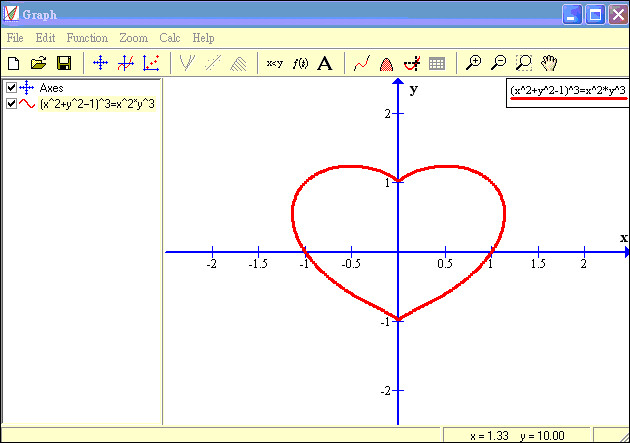This image depicts a computer screen displaying a graphing application. The interface of the graphing software includes a top menu bar with options labeled "File," "Edit," "Function," "Zoom," "Calc," and "Help," in gray letters on a white background. Below this, there are various icons such as a piece of paper, a white folder, a yellow floppy disk, three graph symbols, and magnifying glasses, which are mostly blue, yellow, and gray. 

The main graph area features a heart-shaped diagram in red ink, positioned centrally. The X and Y axes of the graph display numbers ranging from negative to positive values. In the upper right corner of the graph, the formula for the heart shape is displayed, repeating underneath a small box that includes part of the equation, possibly "X² + Y" or a similar mathematical expression. Additional text and checkboxes are visible on the right-hand side of the screen.

The application's interface also has a blue header with the word "Graph" in white letters, next to red and blue line symbols. Icons such as a minimize, maximize, and close button appear in white within colored boxes at the far right of this blue header. Detailed navigation options to adjust the view of the graph are visible, suggesting the ability to zoom in and out and move the graph for closer examination.